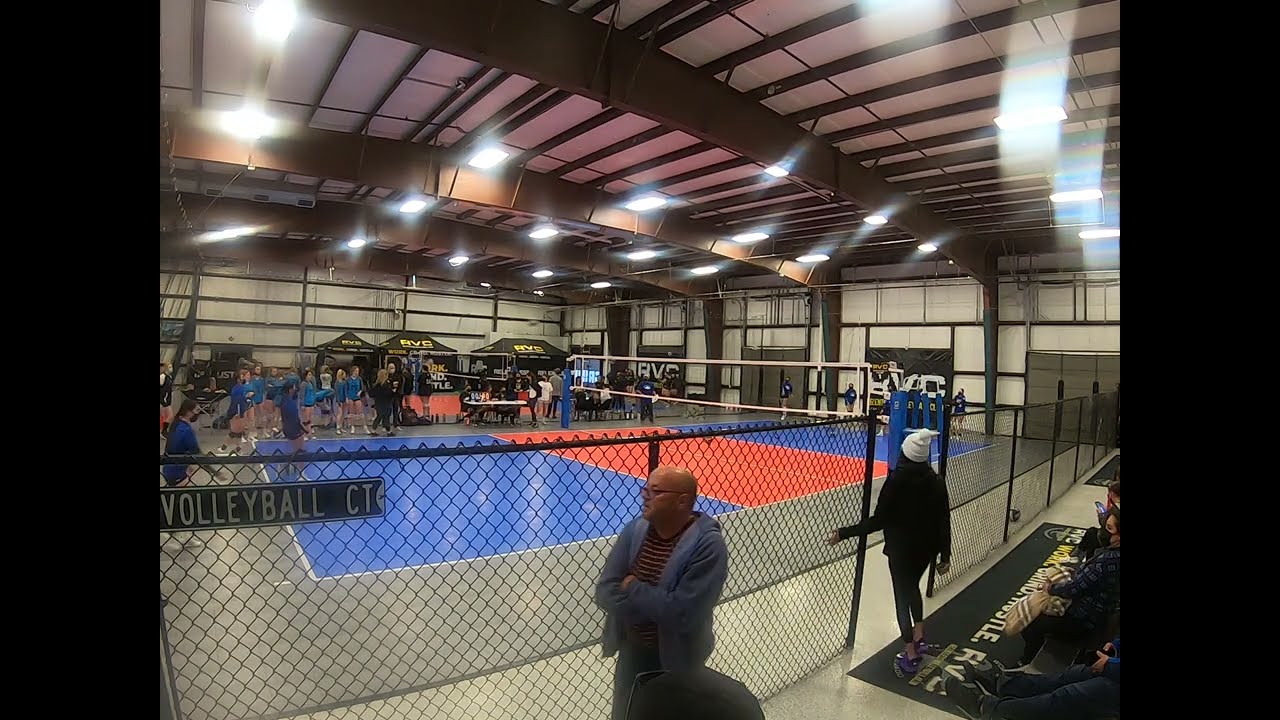This image captures a vibrant indoor scene within a well-lit and clean gymnasium featuring a competitive volleyball match. The focal point is a volleyball court, which is marked with blue and red hues, bordered by a white edge, and divided by a net. Spectators are separated from the court by a black fence, on which a sign reads "Volleyball CT." The ceiling is notably detailed with numerous lights and metal beams, both vertical and horizontal. In the foreground, there's a man standing with arms folded, while other spectators are seated, their legs visible under the fence. Two volleyball teams are seen on the court, distinguished by their uniforms—one in black outfits and the other in blue jerseys with black shorts. In the distance, various tents with letters are set up, and additional people in blue shirts are visible. The gym has white walls with black trimmings, adding to the organized and competitive atmosphere of the ongoing match.